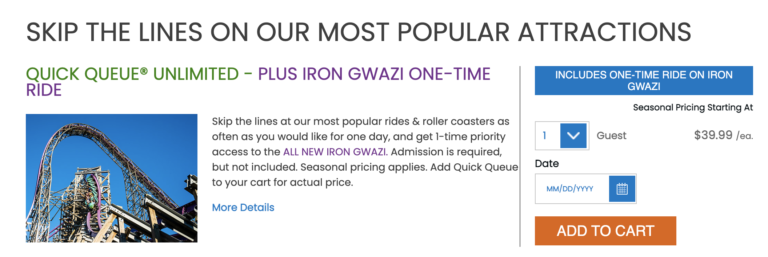Screenshot Description: 

The image is a screenshot of a product offering page focused on ticket options and exclusive access to an amusement park's attractions. At the top of the page, a banner in bold text reads, "Skip the lines on our most popular attractions."

On the left side, there is a segmented section with different offerings. In green, it prominently mentions "Quick Q Unlimited." Adjacent to it, in purple, it states "Bullis Iron Guazi one-time ride."

Below this segment, a vivid image of a roller coaster appears, suggesting the thrill and excitement of the ride. To the right of this picture, there is a text passage providing more details about the offer.

A vertical dividing line delineates two major sections of the page. On the right side of this line, a blue bar highlights "Includes one-time ride on the Iron Guazi." 

Directly beneath the blue bar, text indicates "Seasonal price starting at," followed by a drop-down menu for guests to select their options. To the right of this section, the price "39.99 each" is displayed prominently.

Further down, there is a section for date selection, marked with a blue date picker interface. Finally, at the bottom of the page, an orange "Add to Cart" button invites users to complete their purchase.

The entire page is set against a clean, white background with most of the text in black, ensuring readability and ease of navigation.